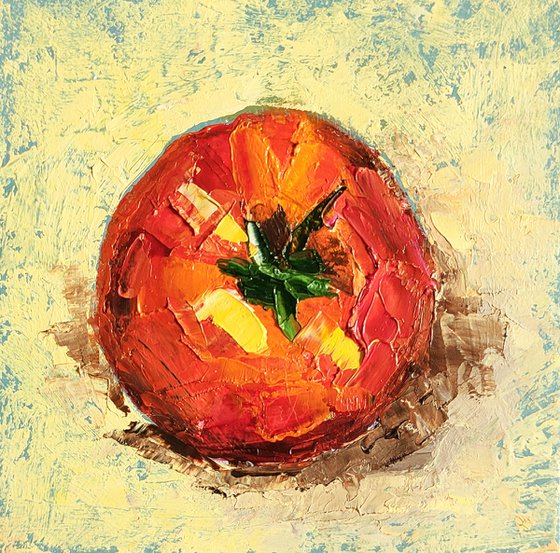The image features a painted tomato viewed from above, set against a soft blue background streaked with a cream color, creating a textured and speckled effect. The tomato itself is a vivid red with patches of yellow, suggesting either unripened areas or highlights from a light source. The green, star-shaped stem sits prominently at the top, where the tomato was once attached to the vine. Surrounding the tomato is a brown shadow that stretches from the middle right to the bottom left, with a small intermittent gap. The painter has used broad, expressive strokes and a generous amount of paint, giving the composition a rich, textured appearance.